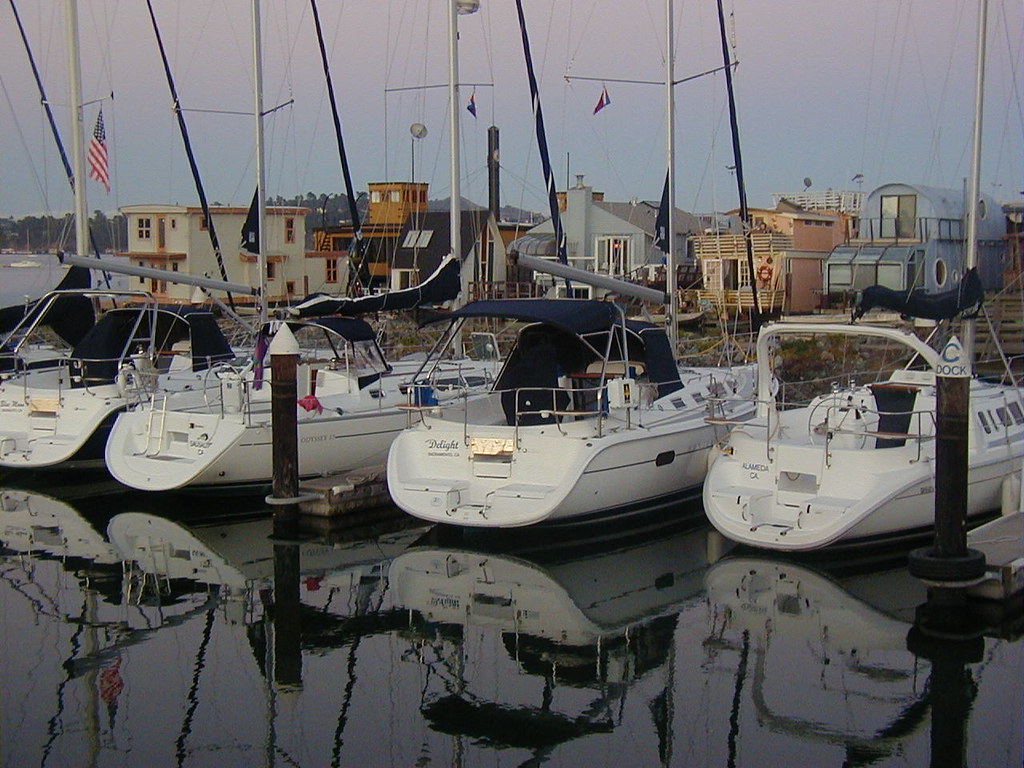This outdoor color photograph captures a serene marina scene at early dawn or dusk, featuring four luxurious, medium-sized sailboats docked with their bows pointing inward. The boats, all sporting white hulls and chrome railings around their sterns, have their masts down and are covered with tarps over the steering areas. The water is remarkably calm, reflecting the boats and the dock structures. On the right, a pole supporting one of the docks bears a blue lettered cap that reads "Sea Dock." The background reveals a row of quaint sea cottages and houses of various shapes and sizes, in hues of blue, pink, and white. An American flag is visible in the upper left corner, fluttering from one of the masts. The docks are anchored by large, thick blackened cement poles, which facilitate the dock’s movement with the tides. The sky, a dark blue with hints of red, adds to the tranquil ambiance of the scene. No people are present on the boats or the dock, and the names on the boats' sterns are not legible.